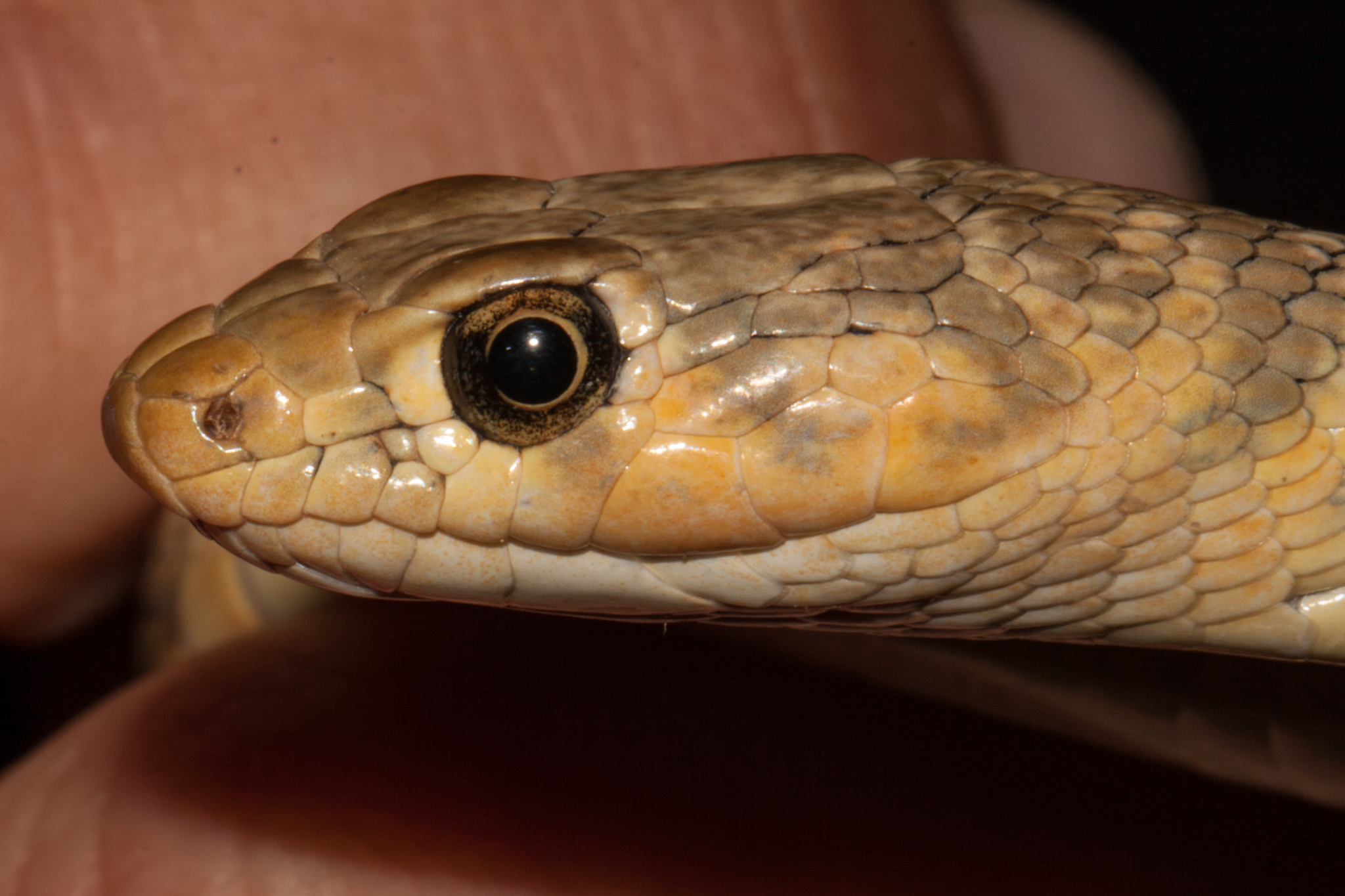The image is a close-up, horizontally aligned rectangular photograph focused on the left side of a snake's face. The snake's head is positioned in the right side of the frame, facing left, and the background is somewhat unclear but includes what appears to be the fingers of a person holding the snake. The snake's closed mouth and intricate scales, which are different shades of brown, beige, orange, and grey, are prominently featured. Its scales have a texture reminiscent of corn kernels. The snake's large, black eye is surrounded by a ring of brown and gold with black speckles in its irises. The coloration is mostly bland, with beige and light orange blending into darker brown tones on the top, and a hint of yellow below the eye. The image is zoomed in so much that it makes the snake appear larger than it likely is, given its potential position on a human hand. Shadows are cast along the bottom of the frame, emphasizing the texture of the snake's head and the close-up nature of the photograph.